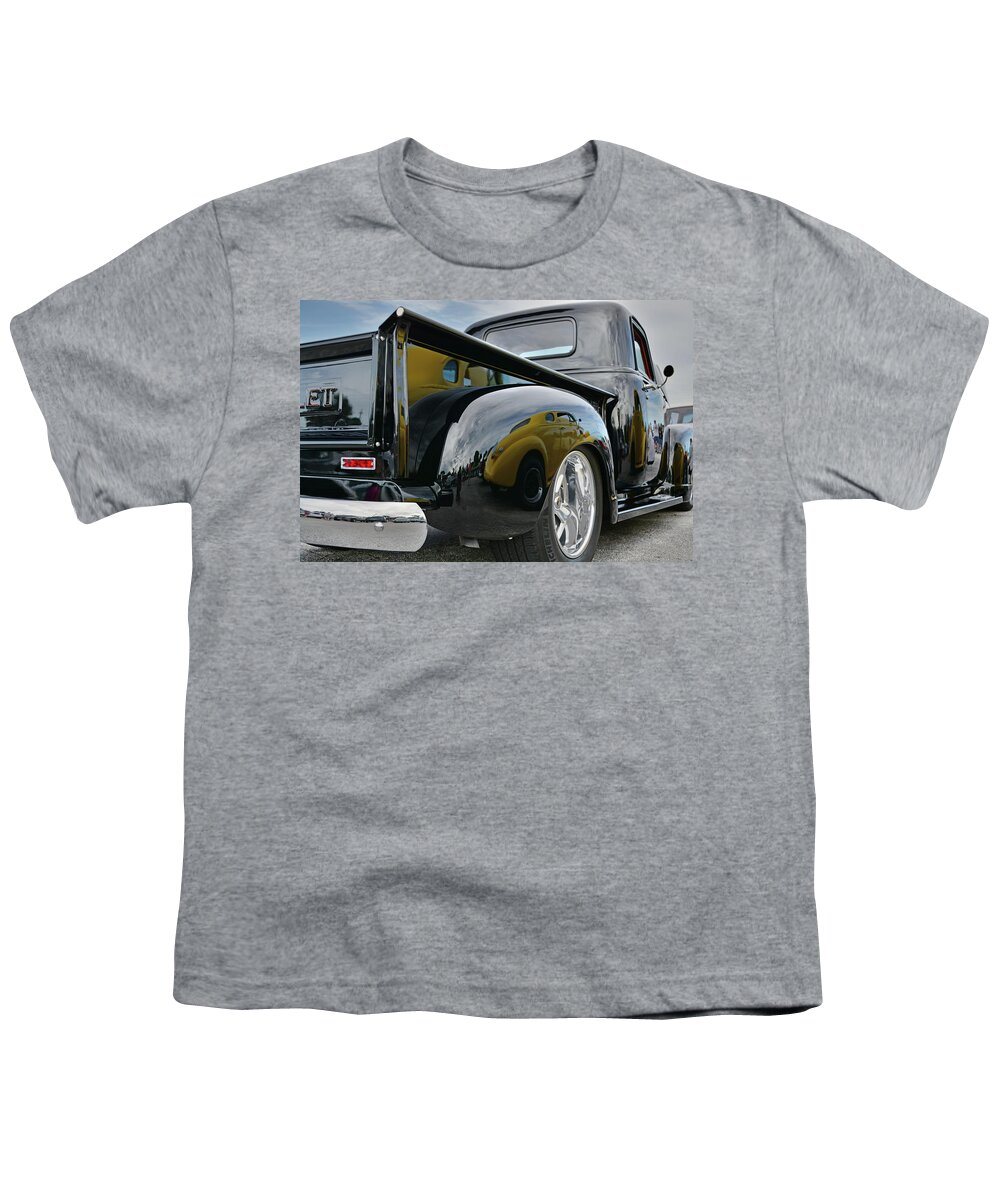The image depicts a gray men's or boy's crew neck, short-sleeved t-shirt, neatly laid flat despite a few ripples around the stomach area. Prominently featured on the front is a horizontally aligned rectangular graphic of a highly polished, vintage black pickup truck, likely from the 1940s or 1950s. The truck's unmistakable shine highlights its freshly painted restoration. The graphic captures the rear and part of the right side of the truck, showcasing a bright silver bumper and large chrome wheels. While no brand is visible on the tailgate, some engraved letters can be noted. The background of the graphic includes a touch of sky, blending shades of gray on the upper right and blue on the upper left. Notably, a reflection of a yellow car can be seen in the truck's finish, adding extra detail to the vintage aesthetic.